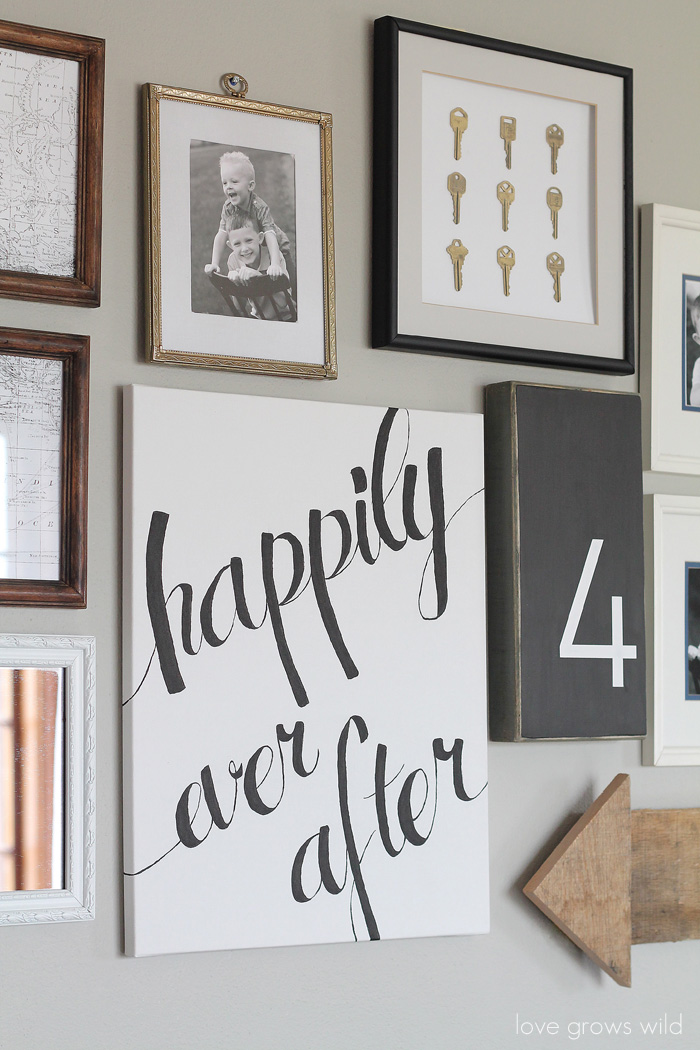The image captures a creatively arranged wall, likely part of a family's home, adorned with a variety of framed pictures, signs, and collectibles against a grey background. Central to the image are different colored and sized frames. Noteworthy items include two vertically stacked wooden-framed maps on the left, a white-framed image of a book, and a gold-framed black and white photograph of two children—one sitting backwards on a chair with the younger child perched on the older one's shoulders.

In the upper right area, a black-framed display holds nine gold keys arranged in a neat three by three grid. Below this display, there's a 3D black box frame showcasing a large white number four. On the bottom left of this area, a wooden arrow points to the left, situated just below a large white poster that reads "Happily Ever After" in black cursive font. Further down on the right edge of the image, one can see parts of two vertically aligned white photo frames. The wall's overall composition exudes meticulous and creative planning, adding a touch of homely charm and personal history to the space.